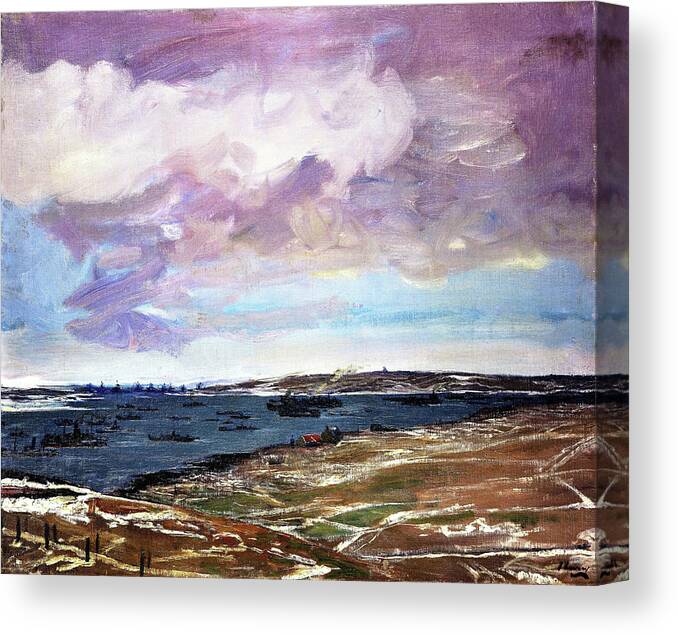The painting, displayed on a square canvas, presents a captivating landscape that transitions from a purple-hued sky with white clouds to a gradient of blue and finally a lighter, whitish sky. The meticulous brush strokes are evident throughout the sky, adding depth and texture. Beneath the sky, the scene reveals rolling hills and a large body of water adorned with various boats and white waves, particularly visible on the left side. The water is dotted with the vague silhouettes of ships, enhancing the sense of distance. The shore is primarily brown terrain interspersed with patches of green grass and streaks of snow. A notable feature is a single red rooftop near the water, standing out against the earthy tones. In the background, there are crisscrossing lines that suggest roads or fences, adding complexity to the landscape. The overall composition intricately blends natural elements with human touches, creating a serene and detailed vista.